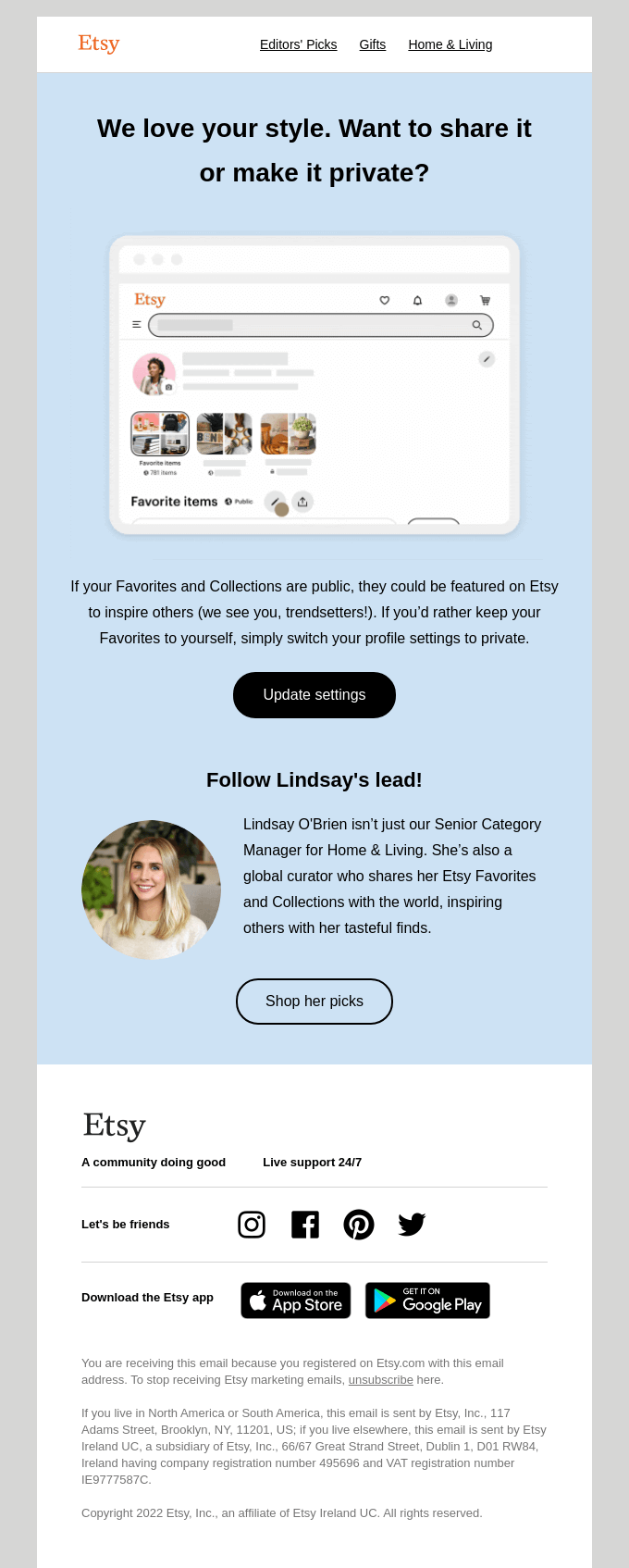The image depicts a webpage from "Earthsea," predominantly showcased in orange. Located at the top left, the "Earthsea" logo is prominent, followed by several navigational categories to the right: "Editor Speaks," "Gifts," and "Home and Living." The main text on the page enthusiastically communicates, "We love your style. We want to share it or make it private." This is emphasized by a central image within the page, embellished with various design elements including a search bar, a magnifying glass icon, the orange "Earthsea" logo, a 'like' button, a notification bell, an 'about you' icon, a cat icon, and several pictures.

Additionally, a notification within the text reads, "If your favourites and collections are public, they could be featured on Earthsea to inspire others. We see you, trendsetters. If you'd rather keep your favourites to yourself, simply switch your profile settings to private." Furthermore, the page invites users to "Update settings, follow Lindsay's lead." Lindsay O'Brien is highlighted as not only the Senior Category Manager for "Home and Living" but also a global curator who shares her Earthsea favourites and collections. Her curated selections are intended to inspire others with her refined taste. The text concludes with a call to action: "Shop her picks."